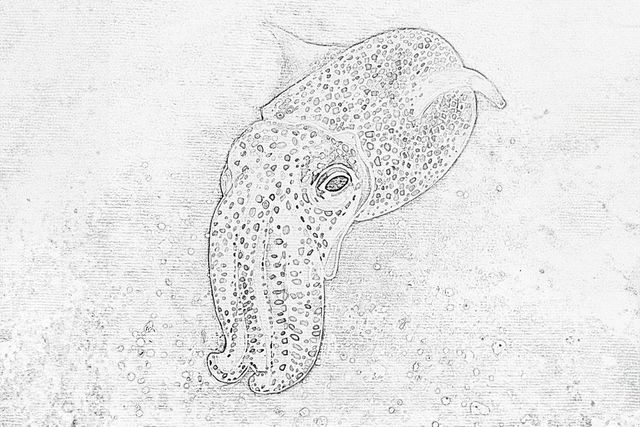This is a detailed black and white drawing of a sea creature resembling an octopus or squid with rich texture and depth. The creature's head is tilted to the left, featuring a prominent left eye and well-defined spots that mimic the texture of its skin. Its body, large and oval, has several fins protruding from the sides. A series of tusk-like structures add to its distinct look. Tangles of tentacles spread out primarily to the left, enhancing the appearance of motion as if the creature is swimming. The background is adorned with a myriad of circular ink marks and splotches, evoking the sense of an underwater environment. Scattered bubbles further suggest that this creature is navigating through the ocean. The use of earthy tones in gray, white, and black highlights the meticulous details of the drawing, emphasizing the organic and lifelike portrayal of this mysterious sea entity.